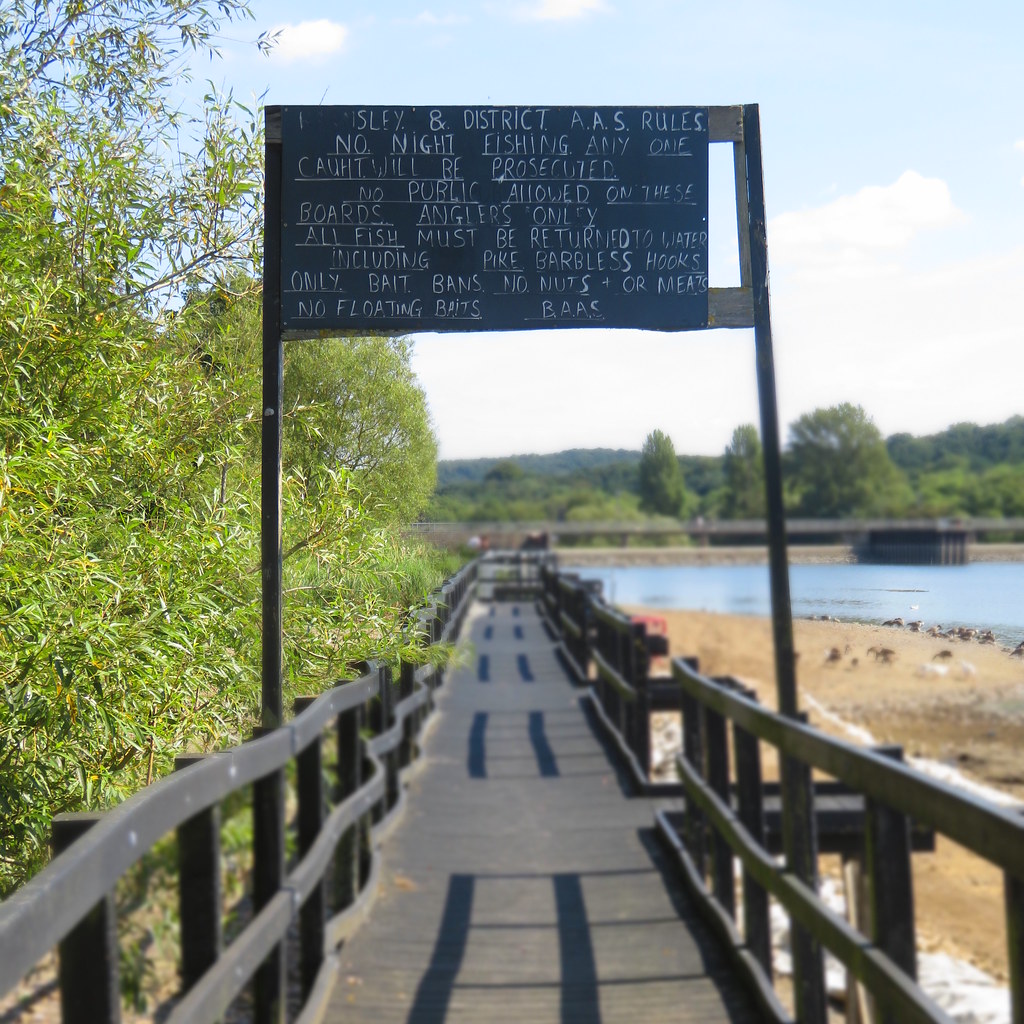This image features a long, narrow boardwalk made of dark, charcoal-colored wood, extending over sandy terrain towards a distant pond or body of water. On the left side of the walkway, trees and greenery are visible, transitioning into more fields and foliage that stretch towards a sky blue horizon with white clouds. To the right, the sand continues, interspersed with birds, leading to a faded blue body of water and possibly a dam or road overpass in the background. Prominently displayed above the boardwalk is a black sign with white chalk writing, outlining strict fishing regulations. Although part of the first word is obscured, the sign reads, "District AAS rules. No night fishing. Anyone caught will be prosecuted. No public allowed on these boards. Anglers only. All fish must be returned to the water, including pike. Barbless hooks only. Bait bands: no nuts or meats. No floating baits." This detailed sign underscores the specific and stringent rules designed for anglers frequenting this picturesque yet regulated fishing spot.